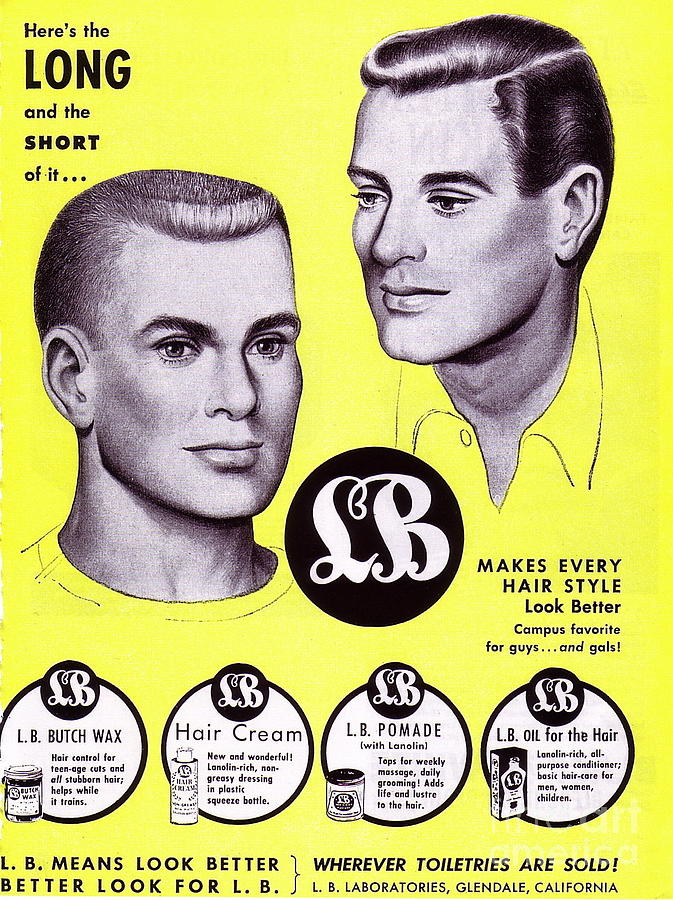The image is a vintage-style advertisement with a predominantly yellow background, featuring black, white, and gray elements. At the top left, in black text, it reads "Here's the long and the short of it." It depicts two men with short hairstyles: one in the top right, facing left, and another in the bottom left, facing down and to the right. A black circle to the right of the bottom left man displays a cursive "LB." To its right, the text says, "Makes every hairstyle look better. Campus favorite for guys and gals." Below, four white circles present LB products, each with a black logo. They advertise: 
1. "LB Butch Wax: Hair control for teenage cuts and all stubborn hair. Helps while it trains."
2. "LB Hair Cream: New and wonderful. Lanolin-rich, non-greasy dressing in plastic squeeze bottle."
3. "LB Pomade with Lanolin: Tops for weekly massage, daily grooming. Adds life and luster to the hair."
4. "LB Oil for the Hair: Lanolin-rich, all-purpose conditioner. Basic hair care for men, women, and children."

At the bottom, it adds, "LB means look better. Better look for LB. Wherever toiletries are sold, LB Laboratories, Glendale, California."